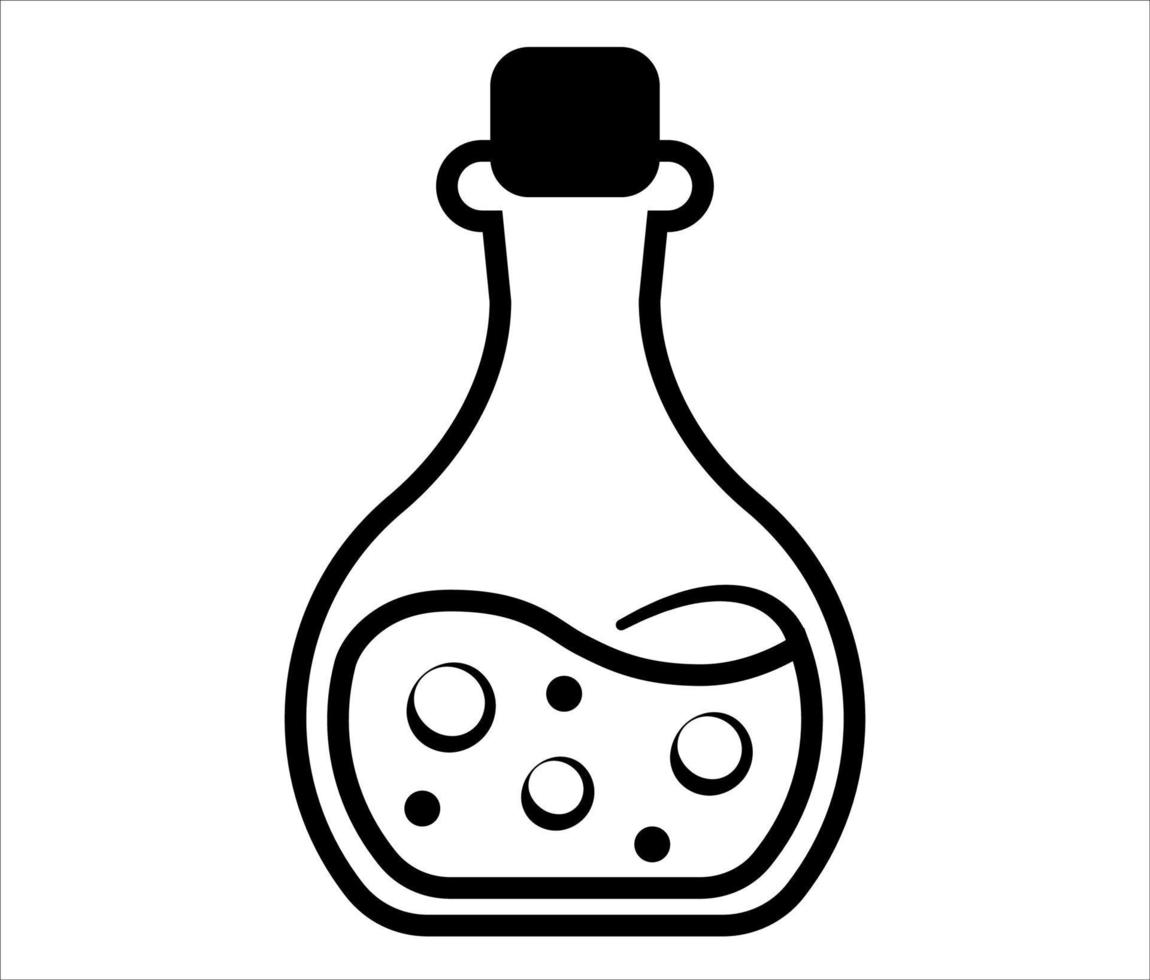The illustration is a black and white line drawing depicting a beaker or potion bottle with a black rectangular stopper at the top. Set on a white background, the bottle displays a black outline. Inside the vessel, which is filled to about a third or half with an unknown liquid, there are detailed visual elements suggesting carbonation or bubbling. Specifically, there are three large white bubbles outlined in black and three smaller solid black circles within the fluid. The liquid level is illustrated with curves, indicating movement or waves. The overall image is devoid of text, people, animals, or any additional background elements, focusing solely on the bottle and its contents.